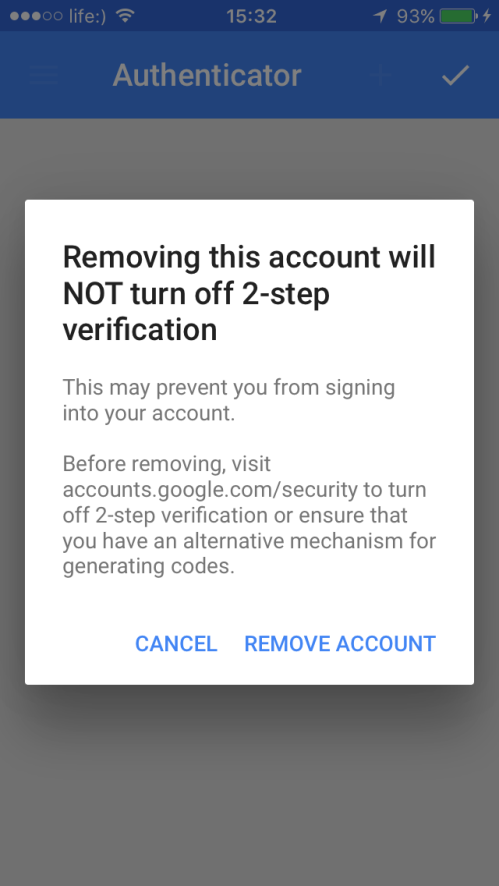In the image, a smartphone screen displays the Authenticator app. The app's header section is blue with the word "Authenticator" written in white on the top-left and a white checkmark on the right side of the header. In the center of the screen, there is a prominent white pop-up notification with black text. The notification reads: "Removing this account will not turn off two-step verification. This may prevent you from signing into your account. Before removing, visit account.google.com/security to turn off two-step verification, or ensure that you have an alternative mechanism for generating codes."

Below this message, two buttons are displayed in blue: "Cancel" and "Remove Account." The general background of the app beneath the pop-up is also white.

At the top status bar of the smartphone, various icons are visible. On the left, the time is displayed as 15:32, and next to it are the Wi-Fi icon and cellular signal strength, which shows three out of five bars. On the right, there is a green battery icon indicating the phone is charging. All these icons are in white, matching the text color scheme of the app header.